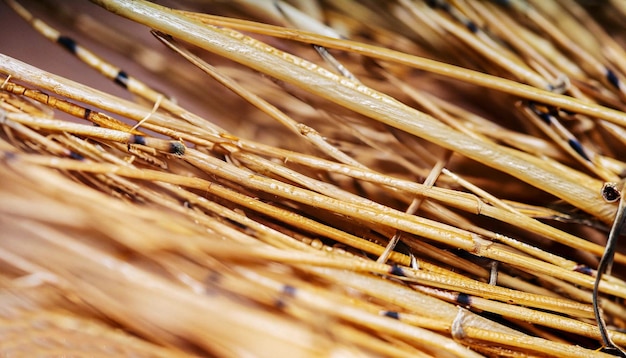This outdoors photograph is an extreme close-up of a bundle of dried grass or hay-like plants, captured with meticulous detail. The stalks, which resemble straw or immature bamboo, are thin and uniformly angled from the top left to the bottom right at approximately a 30-degree angle. The overall color palette consists of golden brown hues with black speckles or stripes intermittently scattered across the stalks, giving them an almost textured appearance. The main focus of the image lies in the middle section, with both the foreground and the background slightly out of focus, creating a depth-of-field effect. The background is notably dark, almost black, further accentuating the dried, straw-like plants. There is no text in the image, allowing the intricate details of the dried stalks to take center stage.